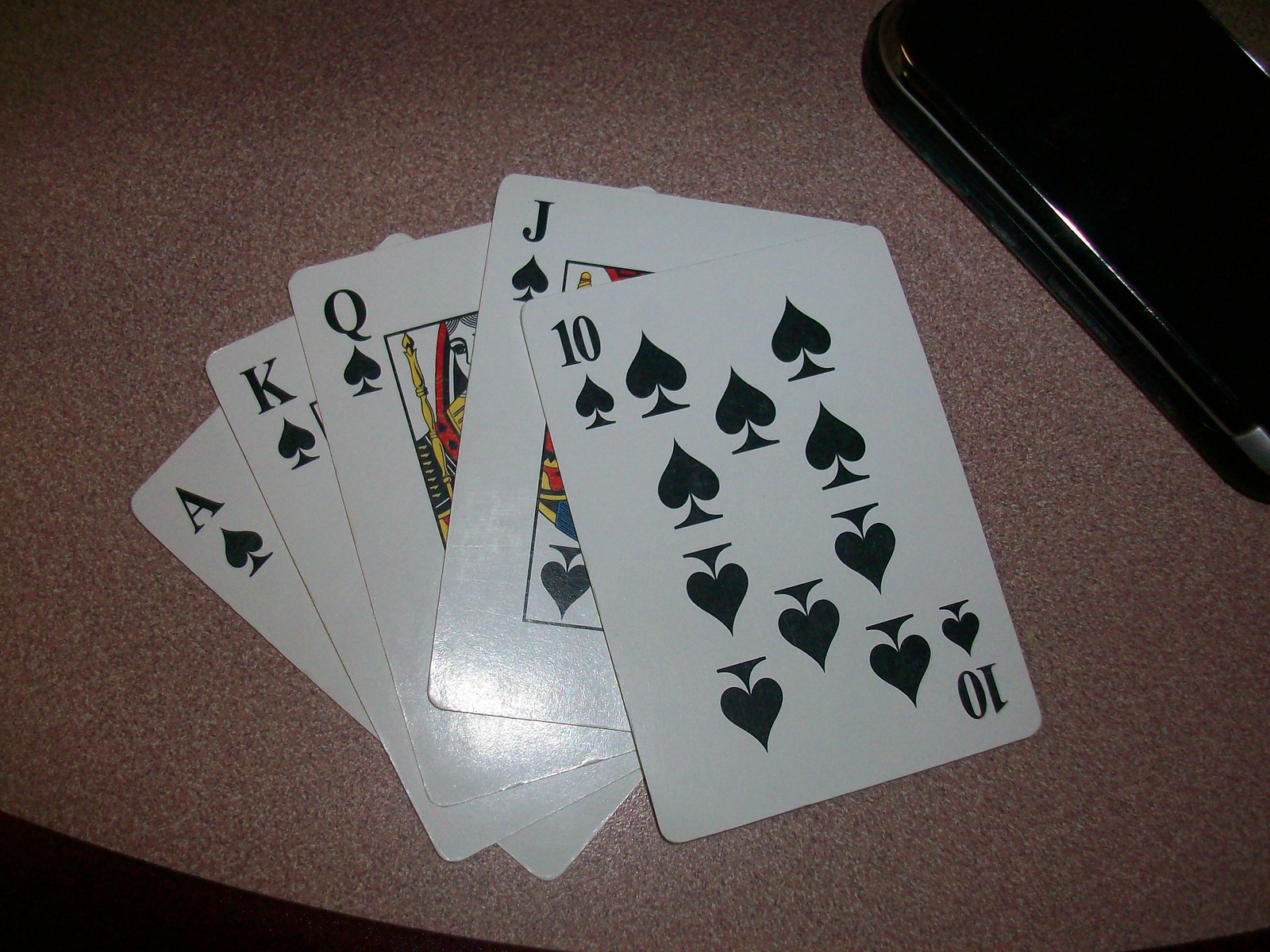The photograph depicts a set of five playing cards prominently displayed on what appears to be a pinkish speckled countertop or desk surface. In the bottom left-hand corner, there is a small triangular area of complete darkness, possibly a shadow or an unlit space. Slightly above this, still in the bottom-left quadrant, the countertop features a subtle pattern of small dots that contribute to its textured appearance.

In the upper left-hand corner of the image, a small black rectangular object rests sideways, its shiny surface reflecting some light. The details of this object are indistinct, rendering its precise function or identity unclear.

At the center of the scene, the five playing cards are positioned in a neatly fanned-out arrangement. The bottommost card, partially visible, is the Ace of Spades, identifiable by its iconic symbol in the upper left corner. On top of this, the King of Spades peeks through, followed by the Queen of Spades whose partial visibility reveals her eye and part of her body. The fourth card in the layer, partially obscured, is the Jack of Spades. Finally, the topmost card, fully uncovered and taking the focal point of the image, is the Ten of Spades, showcasing its complete design.